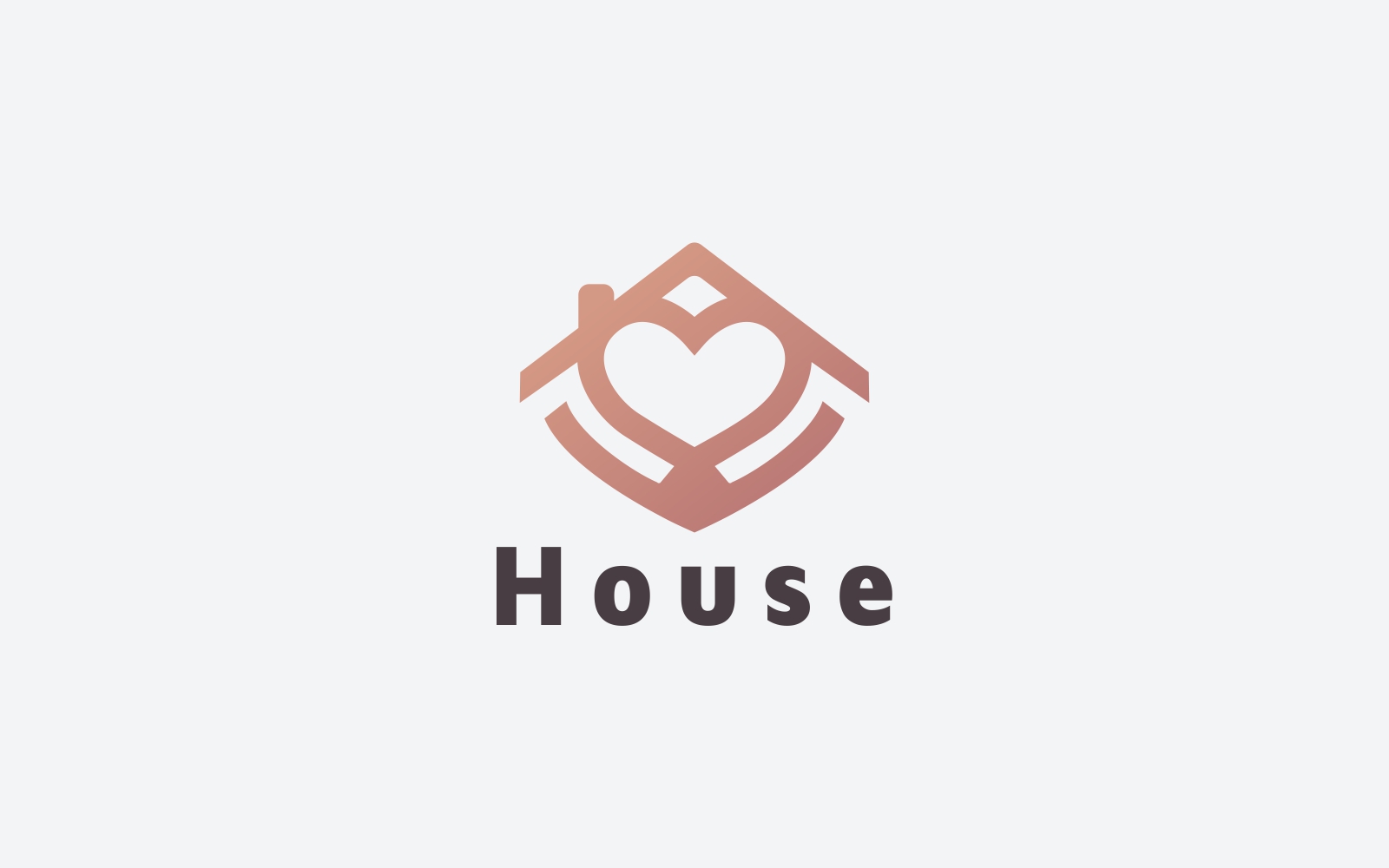The image portrays a minimalist logo consisting of a white or creamy gray background. Central to the logo is a heart icon, prominently positioned in the middle. The heart is encased within an angular design resembling the roof of a house, formed by two slanted diagonal lines: one extending from the bottom left to the top middle, and another from the top middle to the bottom right. A small chimney is depicted on the left side of this roof-like structure. Below the heart and roof design, there is a rounded V-shape that completes the house-like figure. The word "House" is written in spaced-out black letters beneath the icon, giving it a simple, soft, yet effective look. This image likely serves as a logo, possibly for a real estate or home building company, suggesting that they build homes with love as symbolized by the heart.